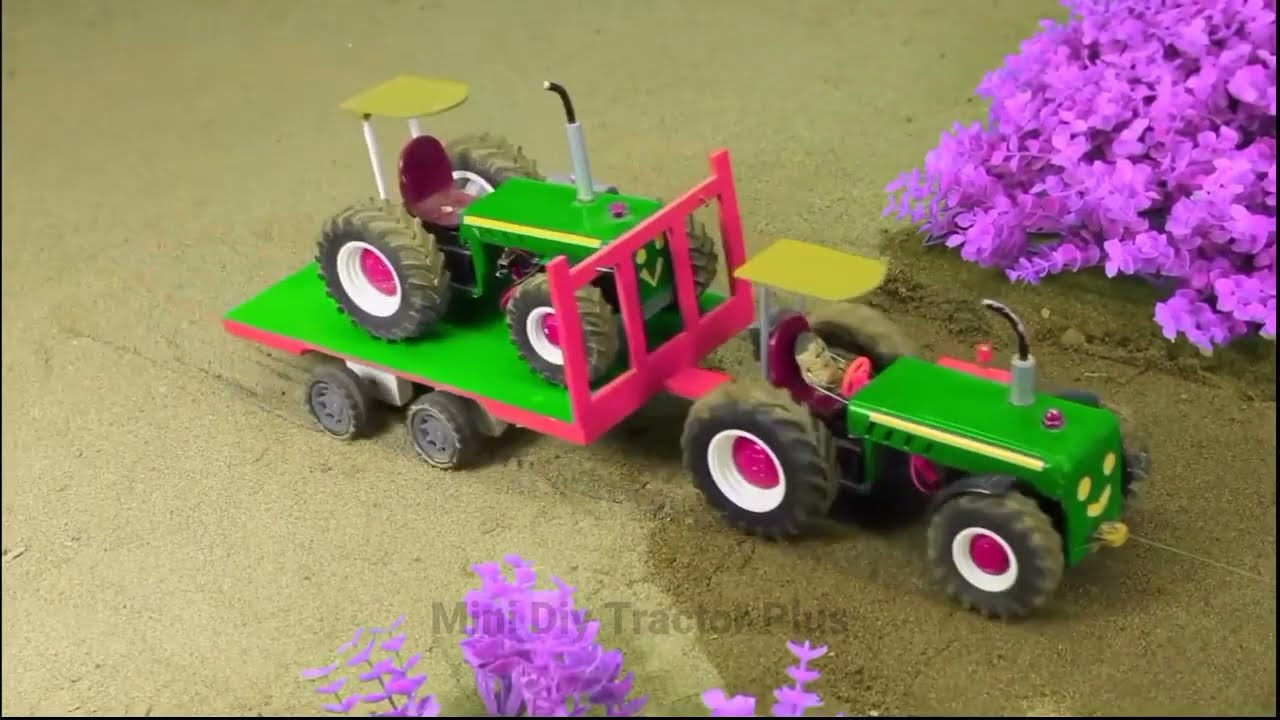In the image, a child's green plastic tractor is featured prominently on a sandy surface, which transitions from dry on the left to wet on the right. The tractor, adorned with a cheerful yellow smiley face on the front, pulls a pink and green flatbed trailer holding an identical green tractor. Both tractors have yellow awnings above their purple driver's seats and sport black tires with white wheels and purple rims. The first tractor is notably driven by a potato figurine gripping a pink steering wheel with its arms. Attached to the front tractor is a piece of fishing line, pulling it towards the right side of the picture. Surrounding the scene are vibrant purple shrubs, located both on the upper right and center bottom of the image. The image also contains text near the bottom that reads "Mini DIY Tractor Plus."